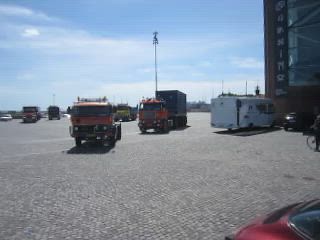This photograph captures a sprawling outdoor parking lot, seemingly a truck stop, filled predominantly with various large trucks. The lot itself has a bumpy texture with a surface made of concrete or gravel. At the center of the image stands a vertical sign that reads "parking." Prominently, two orange big rigs are parked diagonally, facing the camera. To the right of these trucks, a white RV is positioned, facing a tall structure that could be a parking building or a large telephone pole. Additional vehicles include a black car and the front wheel of a bicycle near the RV. Closer to the viewer, the back of a red sedan is visible. The sky is bright blue, adorned with a few fluffy, ethereal clouds, hinting it could be around mid to late afternoon. Overall, the image teems with a mix of heavy-duty trucks, smaller cars, and a backdrop of infrastructure, epitomizing a bustling truck stop scene.